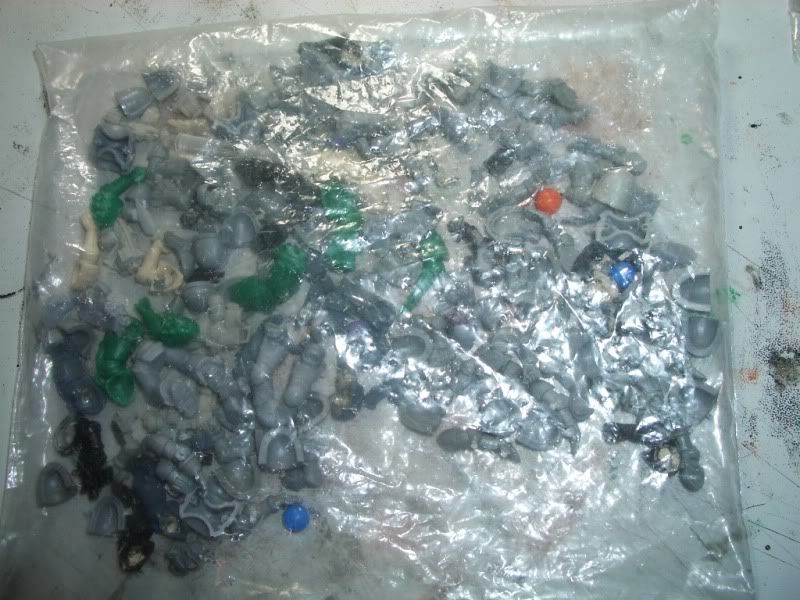The close-up image captures a reflective plastic bag filled with numerous small, gray parts that vary in size and shape. Scattered among these predominantly gray pieces are a few green parts on the left side, along with a couple of blue ones and a single orange piece interspersed throughout. The bag features white lettering that reads "Photobucket" next to a circular design with concentric circles. Below this, a slogan proclaims, "Protect more of your memories for less!" The reflective quality of the bag causes bright light to obscure the visibility of the parts inside. The bag is resting on a white surface that shows signs of wear, with scratches and scuff marks visible around its edges. On the right side of the image, distinct scuff marks can be seen—one green and one orange—alongside some black marks and a black circle.